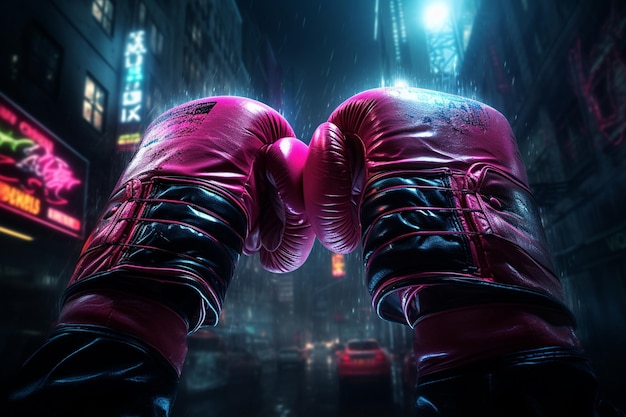The image is a highly detailed, likely AI-generated, artistic rendition of two boxing gloves held high in the air, positioned centrally in the frame. The gloves, which are futuristic and colored in vibrant purple and black shades, are shiny and reflective, capturing the gleam of city lights. The scene showcases a narrow, rain-soaked street at night, flanked by tall buildings adorned with neon signs and banners, some displaying Japanese characters. The street is lively, with cars driving through and their headlights visible, further accentuating the night-time atmosphere. The background is a bustling urban landscape, featuring neon-lit signs that add a touch of color and modernity amidst the dark, bluish hues of the rainy night. Water droplets are visible on the gloves, enhancing the realism and moodiness of the scene, while the rain continues to pour, making the entire composition dynamic and immersive.